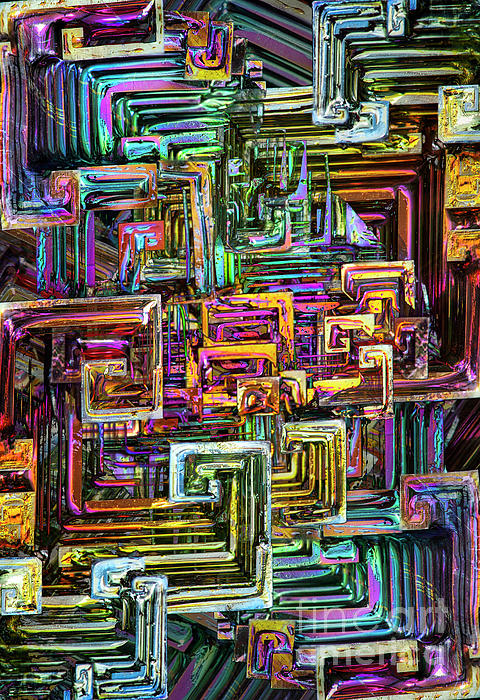This painting is a vibrant and intricate piece of abstract art, bursting with virtually every color imaginable. The artwork features a plethora of geometric shapes and patterns, including numerous interconnected L-shaped forms, arches, and what appear to be staircases seen from an aerial perspective. These shapes are present in a wide spectrum of colors such as pinks, blues, greens, golds, yellows, oranges, and purples, often neon-bright, creating a dynamic and modern aesthetic. The colors blend and overlay each other, contributing to a complex, 3D-like effect. The composition of the painting draws the eye towards the center, with the shapes mirroring and leading into one another, generating a sense of depth and continuity. At the very bottom, written in faint, white text, is a watermark that reads "fine art," with an additional word that is difficult to decipher due to its subtle overlay on the vibrant background. This captivating piece would make a striking focal point on a white wall, adding a splash of vivid color and contemporary flair to any space.